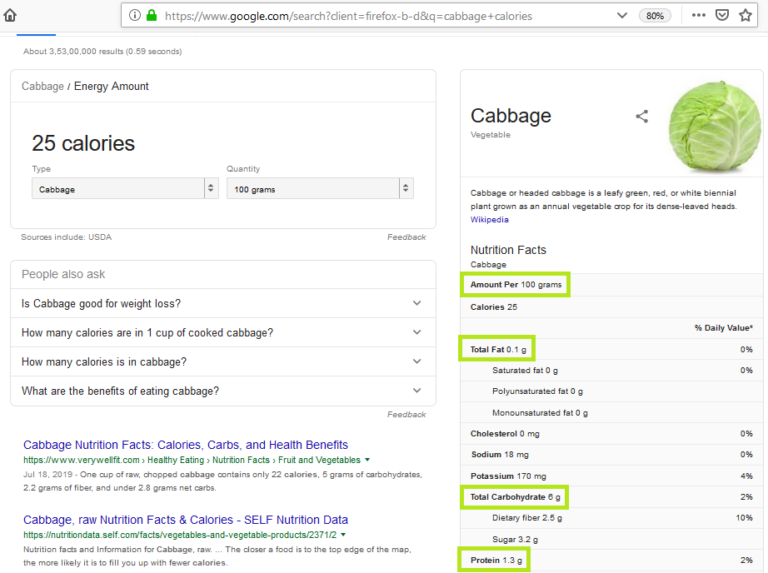The image displays a web page with a search result for "calories in cabbage" on Google. At the top of the page is a home icon, and a search bar containing the query. The search result indicates that 100 grams of cabbage contain 25 calories. It cites the USDA as a source and includes feedback options. Additionally, there are related questions listed, such as "Is cabbage good for weight loss?", "How many calories are in a cup of cooked cabbage?", and "How many calories in cabbage?".

On the right side of the page, there is an image of a green, round head of cabbage, displaying the veined leaves. Accompanying the image is text from Wikipedia describing cabbage, or headed cabbage, as a leafy green, red, or white biennial plant grown as an annual vegetable crop for its dense-leaved heads.

Below this, there is a section showing nutritional facts bordered in green. It indicates that cabbage has 0.1 grams of total fat and 0 grams of potassium tetracarbohydrate, highlighted with a lime green border. The overall layout provides detailed nutritional information about cabbage.